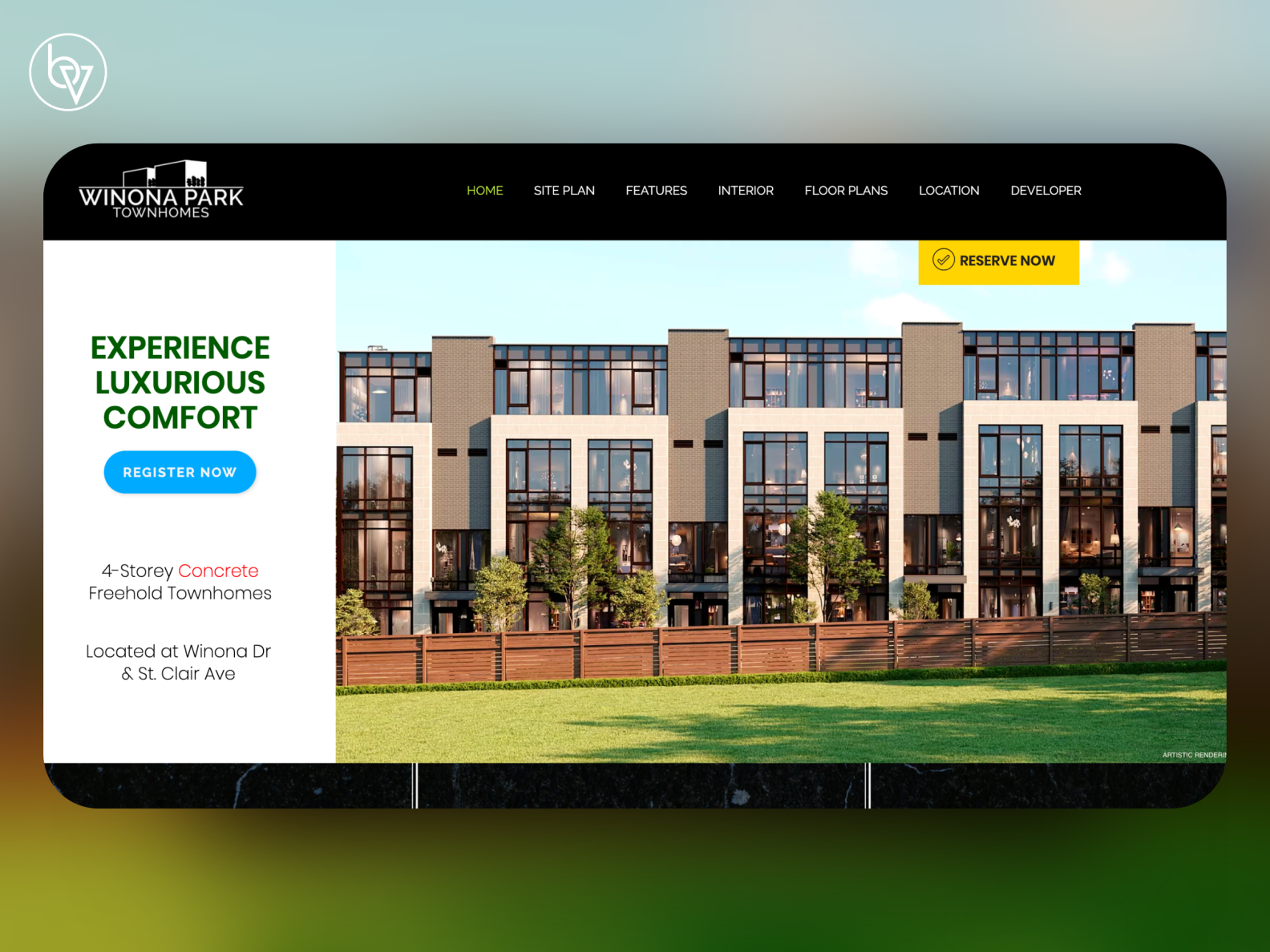The screenshot captures the landing page of Winona Park Townhomes. The header features a sophisticated black background with smooth, rounded corners rather than sharp edges. On the far left side of the header, "Winona Park Townhomes" is prominently displayed in white text, accompanied by a logo depicting abstract black and white box-like buildings.

The navigation tabs within the header include options labeled Home, Site Plan, Features, Interior, Floor Plans, Location, and Developer.

The central image displayed on the webpage showcases a modern architectural design of the townhomes. These buildings have a flat rooftop and extensive glass walls, reflecting a contemporary and clean aesthetic. The design is further characterized by distinctive white sections with an inverted U-shape pattern. Surrounding the building is a stylish white wooden fence, complementing the sleek appearance. In front of this fence, there is a well-maintained, flat expanse of green grass.

On the left side of the webpage, occupying about one-fourth of the screen, is a white section with the text: "In Green Experience, Luxurious Comfort." Below this, a blue "Register Now" button invites visitors to take action. The section also includes two lines of text describing the property: "Four-Storey Concrete Freehold Townhomes located at Winona Drive and St. Clair Avenue."